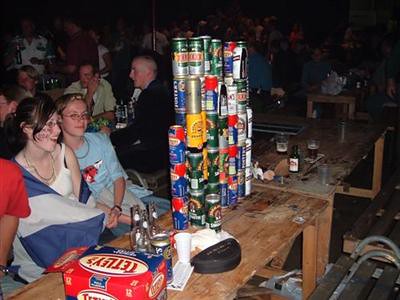The image captures a lively scene at what appears to be an outdoor festival, possibly the Glastonbury Festival, given the muddy surroundings and the festive atmosphere. Wooden tables, marked by years of wear and tear, are laid out in a communal fashion with scattered beer cans, some creatively stacked into a tower formation. It’s unclear whether these cans are full or empty, but a box of Tetley's beer is prominently placed on one of the tables.

In the dim lighting, people are seen congregating and enjoying their time, their silhouettes and the occasional glint off a bald head who appear among the chatting crowd. A notable table shows two women engaged in conversation. One of them wears a blue short-sleeve shirt, a black watch on her left wrist, and glasses, her blonde hair catching the sparse light. Beside her sits a woman with brown hair pulled into a ponytail, dressed in a white tank top and adorned with a necklace. She notably has a blue and gray flag draped around her shoulders. The table in front of her is cluttered with two empty beer bottles and the Tetley's box. Despite the darkness, the camaraderie and enjoyment of the gathering are palpable.